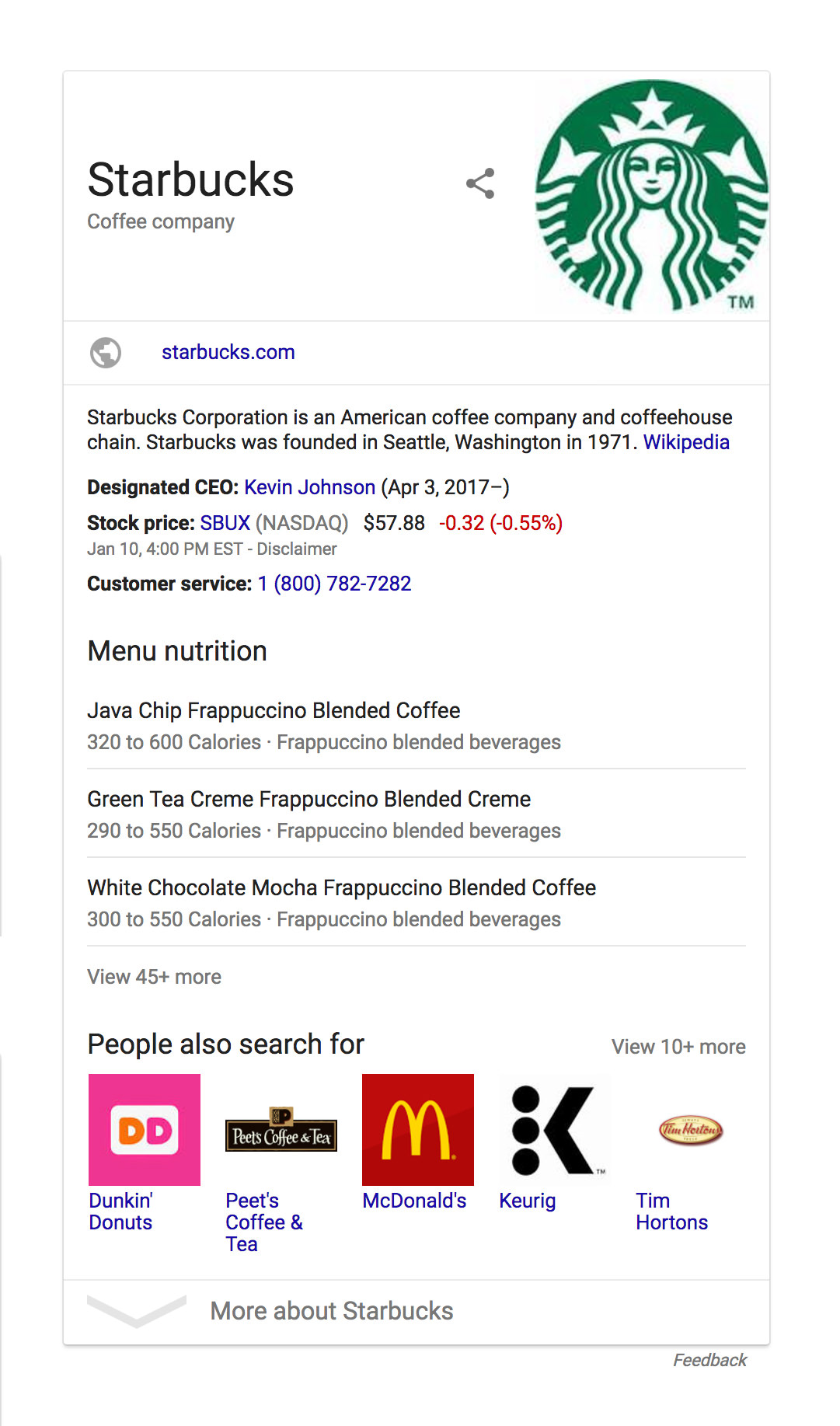This image is a screenshot taken from a mobile phone, displaying the Starbucks Corporation page, likely from a search engine or informational website. At the top of the screen, the word "Starbucks" is prominently featured in black print, followed by "Coffee Company." In the far-right corner, the iconic green and white Starbucks logo is visible, depicting a mermaid figure with long flowing hair, a crown with a star above it, and a "T.M." mark in green at the edge.

Beneath the company name, the URL "Starbucks.com" is shown, followed by a brief description: "Starbucks Corporation is an American coffee company and coffeehouse chain. Starbucks was founded in Seattle, Washington, in 1971," attributed to Wikipedia. Additional details include the name of the CEO, Kevin Johnson, with his tenure starting from April 3, 2017, onward. 

Further down, the page displays stock price information, customer service contact details, and sections on the menu and nutrition. Specific menu items like the Java Chip Frappuccino Blended Coffee and Green Tea Cream Frappuccino Blended Cream are listed with their calorie counts, ranging from 320 to 600 for the Java Chip Frappuccino. The white chocolate mocha Frappuccino's calorie content is also mentioned.

At the bottom, there is a "People also search for" section, presumably listing other relevant companies or topics related to Starbucks. The overall layout and information suggest that this screenshot provides a comprehensive overview of Starbucks' corporate and nutritional information as found online.